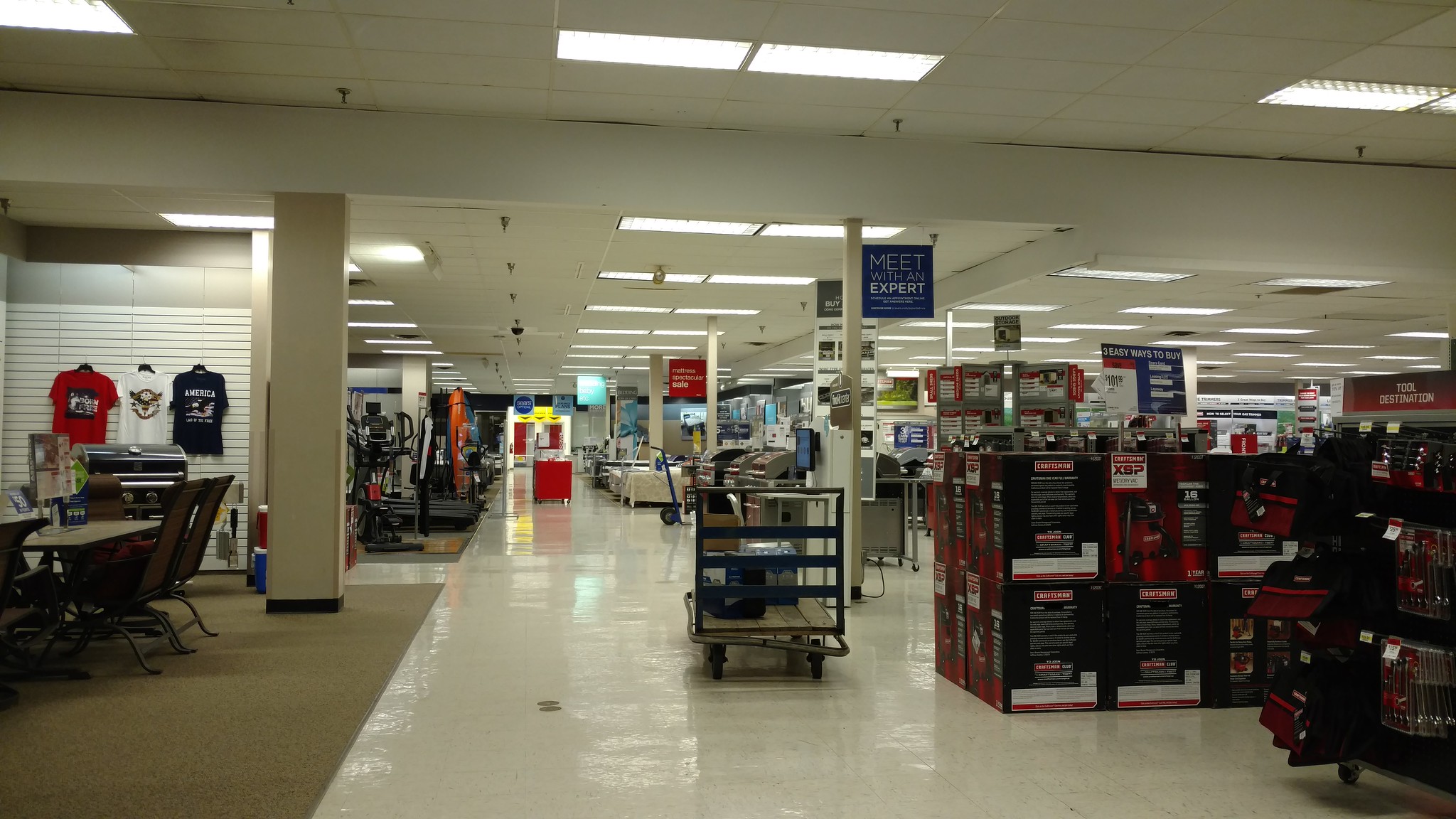A detailed caption for the image could be:

"The image depicts the interior of a well-lit department store with a glossy white tiled floor and carpeted areas designating different sections on the left. Prominently on the right, there are black and red boxes, though their contents are not identifiable. Centrally located is a wheeled cart, possibly used by a worker or shopper, although no individuals are present in the image. The depth of the store is evident as it stretches far back, showcasing numerous columns and ceiling-hung signs that invite customers to 'meet with an expert.' On the left, three shirts are displayed on a wall above a table that resembles a grill, suggesting a campsite setup. Further back on the left side, various pieces of exercise equipment are visible. The ceiling is adorned with an array of lights, illuminating the entire space."